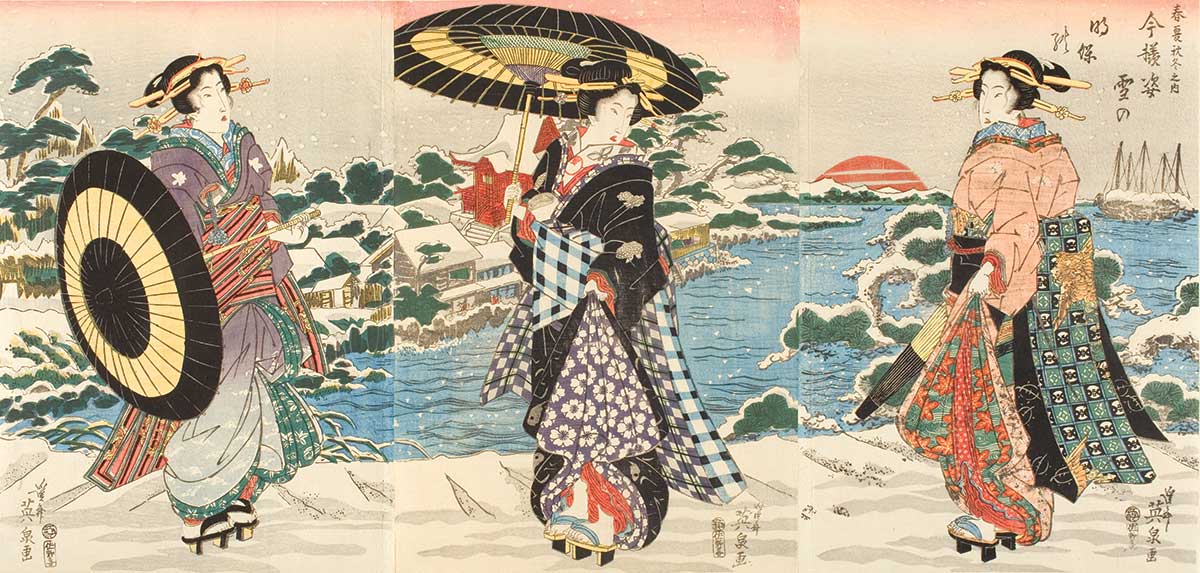The image is a detailed triptych, depicting a traditional Japanese winter scene with three elegantly dressed geisha. They stand on a snow-covered path beside a serene body of water, over which a red sun rises, casting a soft pink hue across the sky. Snow blankets the trees, shrubs, and roofs of a small village and a red pagoda visible in the background. The geisha wear ornate, colorful kimonos and obis, adorned with intricate patterns and accessories, including geta sandals and hairpins. The woman on the left, in a purple dress with red and black striped sashing, holds her parasol sideways as if spinning it. The central figure, dressed in a black kimono with a red and white top and a purple, paisley-flowered layer, holds her open parasol above her. The woman on the right, wearing a salmon-colored top with a green and red floral train, carries her folded parasol and what appears to be a bag. Japanese characters grace the upper right and bottom edges of the painting, enhancing its traditional aesthetic.